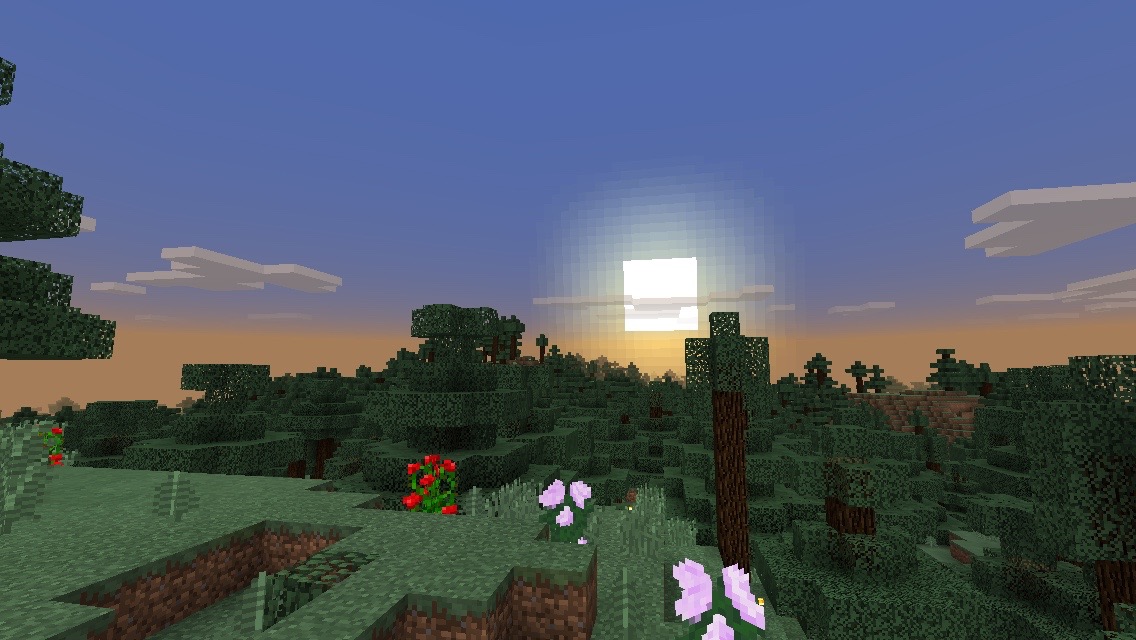This artwork, which could be a drawing, lithograph print, or painting, presents a captivating and highly stylized scene. Dominating the upper half of the image is a bright blue sky adorned with a few distinctly stylized clouds. These clouds are angular and appear as light gray slabs, starkly contrasting with the typical fluffy forms we expect. The sun takes on an unconventional, square shape, resembling a brilliant mirror suspended just above the horizon.

The trees in the scene also deviate from naturalistic representation; they exhibit a boxy appearance with sharp, angular limbs, though they are rendered in various shades of green. This geometric, almost mechanical portrayal extends to the lawn in the lower left-hand corner. The grass is a uniform green but interspersed with small, boxy shapes, contributing to the overall abstract aesthetic. This meticulous arrangement of angular elements and vibrant colors produces a unique, thought-provoking composition, rich in detail and creative expression.